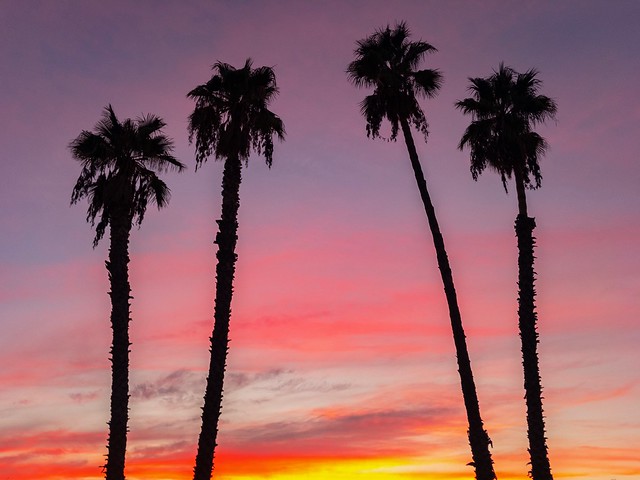An outdoor sunset scene features four silhouetted palm trees with tall, bare trunks topped by lush fronds. The trees are positioned with two on the left and two on the right, creating a balanced focal point against a colorful sky. The sky transitions from a deep purple at the top to pink in the middle, and finally to vibrant hues of yellow and orange near the bottom, suggestive of the setting sun just below the horizon. Wispy grayish clouds catch the last light, turning pink as they ascend. The tallest tree is the third from the left, and all the trees stand starkly against the backdrop, enhancing the dramatic contrast of the scene.